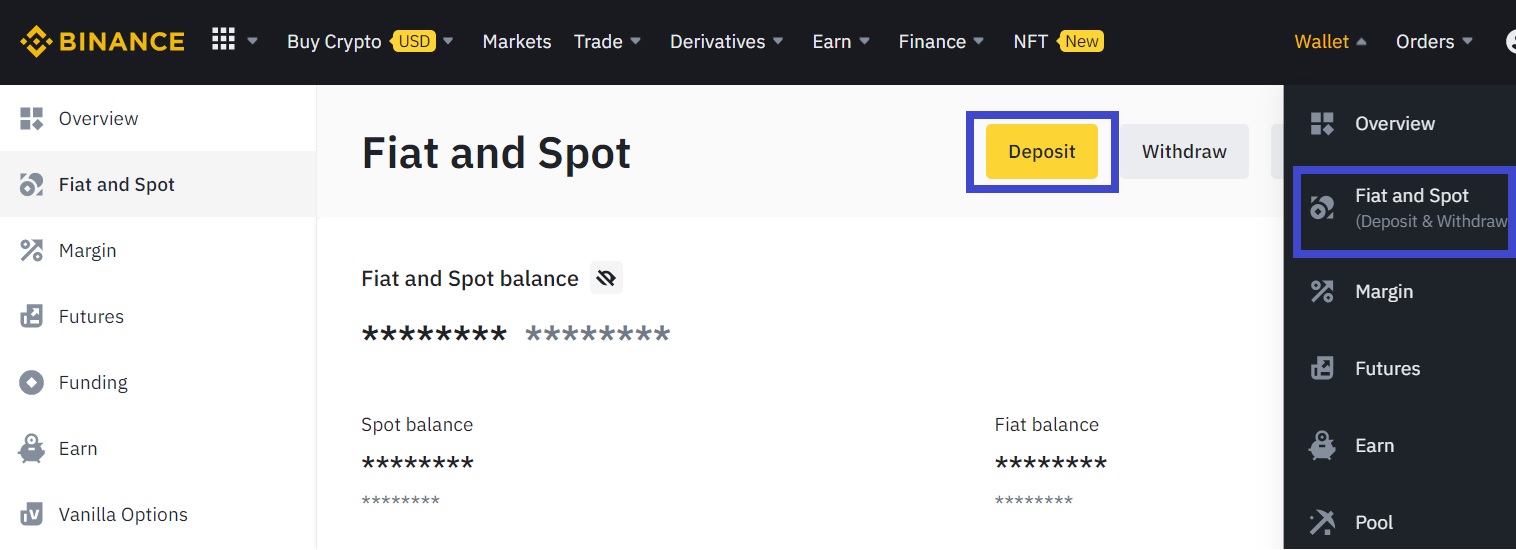The image is a screenshot of the Binance website interface on a desktop screen. At the top, there is a black header section displaying the yellow Binance logo along with the company's name. To the right of the logo, there are several menu options in white text: "Buy Crypto," which has a black drop-down arrow, followed by "USD" written in black ink over a yellow background, also accompanied by a gray drop-down arrow.

Continuing along the header, there are additional menu options: "Markets," "Trades," "Derivatives," "N," "Finance," and "NFT," each featuring a gray drop-down arrow. "NFT" also has the word "New" highlighted in black ink on a yellow background. Toward the end of this header menu, there are sections for "Wallets," which includes a yellow icon with an upward-facing arrow and "Orders" in gray text.

Below this header, the image showcases various sections of the Binance interface. There is an "Overview" segment for wallets, "Fiat and Spot" with a blue border, followed by categories such as "Margin," "Futures," "N," and "Pool". Each of these sections is laid out on a predominantly white background. Adjacent actions such as "Deposit" and "Withdraw" are also visible in the interface.

Overall, this detailed screenshot provides an extensive overview of Binance's homepage layout, featuring multiple financial menus and functionalities designed for users of the cryptocurrency platform.